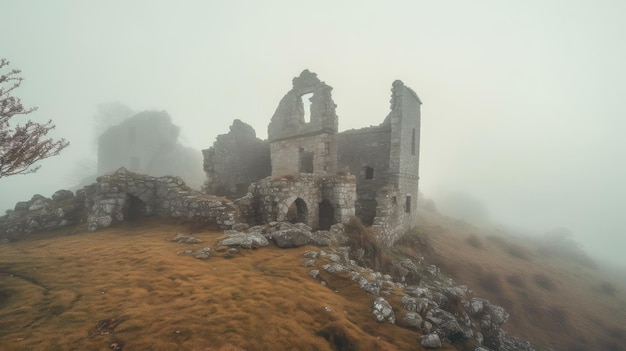In this image, we observe the ruins of what appears to be an ancient castle or stone building situated on a mountainous terrain. The ground is adorned with orange and brown hues, reminiscent of dead grass and a barren hillside, interspersed with scattered rocks. The remnants of the structure suggest it once featured windows and walls, though now only a small, prominent portion of the stone edifice remains standing. The scene is shrouded in a dense, foggy atmosphere, with a predominantly cloudy sky allowing glimpses of blue. The left side of the frame includes a partially visible tree with brown leaves, enhancing the image's somber, desolate mood. In the misty background, additional hills and hints of more ruins or rocky formations are barely discernible, amplifying the sense of an abandoned and decayed historic site.